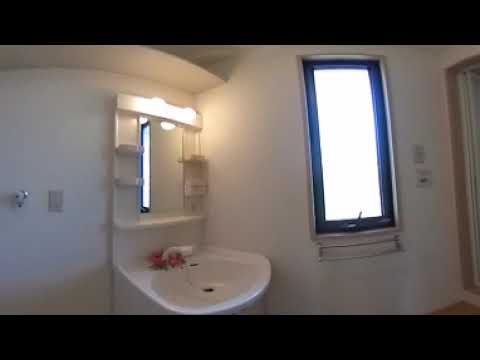A captivating panoramic photograph, resembling the view through binoculars or a convex viewfinder, captures a scene divided into three distinct sections framed by metallic outlines. The central section showcases a vibrant field with green grass and a hill adorned with lush trees in the background to the right. Above this serene landscape, a blue sky is scattered with white clouds. Scattered buildings lie in the distance, further enriching the scenery.

To the left of this central vista, a man dressed in a white button-down shirt and black pants stands within what appears to be an enclosed area of a building or possibly the connecting space between two train cars. This man, likely of Asian descent, is holding a selfie stick, suggesting he is taking a photo of the scene. He stands near a sliding glass door, which might be an entry into a train car or a balcony area.

On the right, a smaller, partially visible section reveals an arm and a hand, likely belonging to the man on the left, with hints of the train car's interior, including a window and the flooring. This section cuts off abruptly, leaving only glimpses of the enclosed space beyond.

Overall, the image offers a dynamic blend of natural beauty, human presence, and architectural elements, all framed by the metallic borders reminiscent of a viewfinder, suggesting a panoramic journey through both landscape and structure.